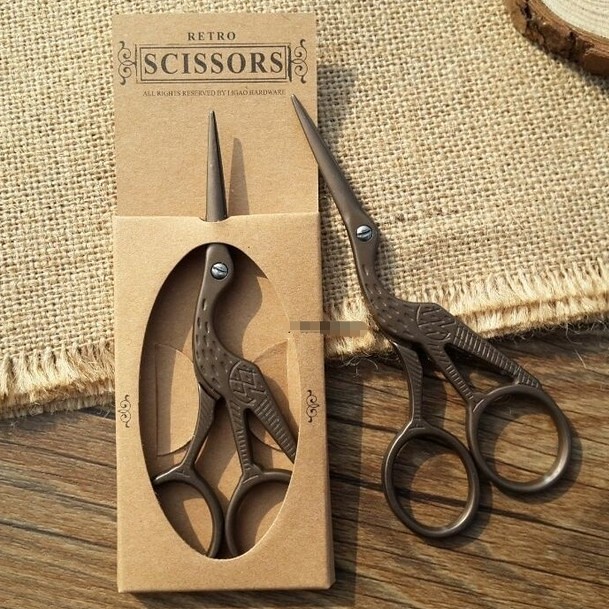This image features two pairs of intricately designed scissors, both emphasizing a vintage aesthetic. The scissors have unique, bird-like handles with a curved design that resembles a bird with three legs, a pointed beak, and a silver screw functioning as an eye. One pair of scissors is displayed inside a cardboard packaging labeled "Retro Scissors" with additional, partially visible text that may read "all rights reserved" and reference something hardware. The packaging features an oval window, making the scissors’ distinctive shape visible from the outside. The second pair of scissors lies outside the packaging, to the right of it. Both the boxed and unboxed scissors rest on a medium brown wooden table with a portion of the scene overlapping onto a quilted beige blanket or tablecloth. At the top of the image, there is a round, wooden coaster made from a tree slice, adding a rustic touch to the setting.